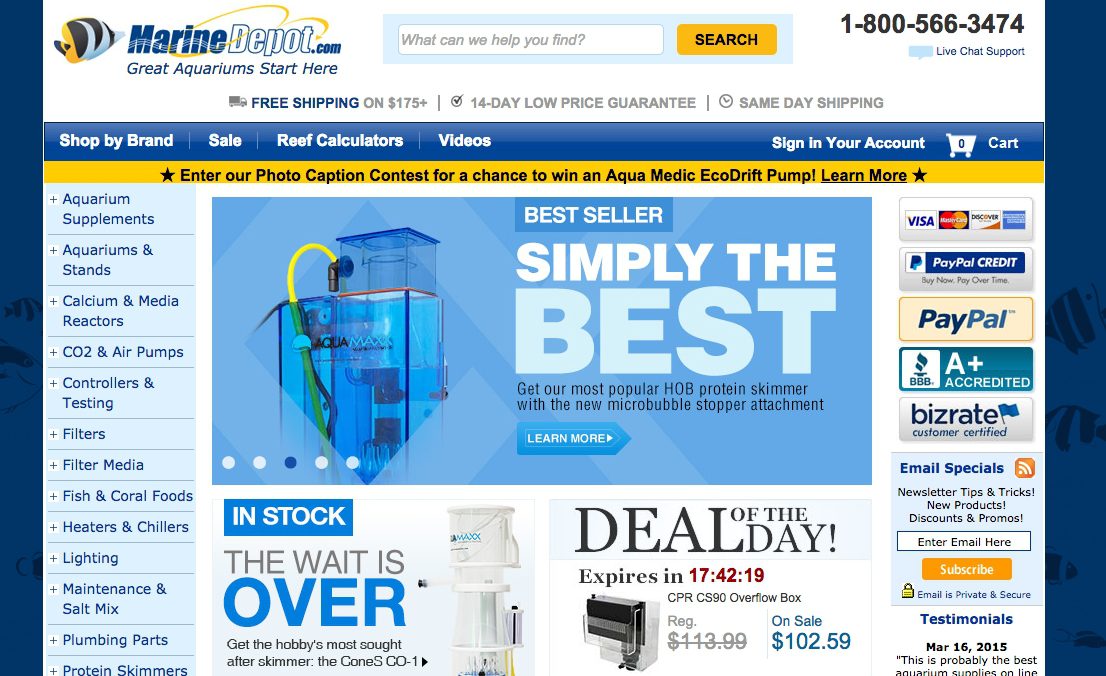The homepage of MarineDepot.com welcomes visitors with a prominent headline: "Great Aquariums Start Here." A search bar sits centrally, featuring a bright orange search button. The top of the page displays a customer service phone number, 1-800-566-3474, and offers live chat support. Visitors are enticed with promotional highlights including free shipping on orders over $175, a 14-day low-price guarantee, and same-day shipping.

The navigation menu allows users to shop by brand, explore sales, access reef calculators, and watch videos. Personalized options are available, such as signing into your account and viewing your cart. A highlighted promotion invites users to enter a photo caption contest for a chance to win an AquaMedic EcoDrift pump, with a "Learn More" button for additional details.

Dominating the center of the page is a large blue banner advertisement. It features an announcement for their best-selling product: the highly popular HOB protein skimmer, now available with a new micro bubble stopper attachment, along with another "Learn More" button. To the right, a countdown timer urgently showcases the "Deal of the Day" on a CPR CS 90 Overflow Box, currently set to expire in 17 hours, 42 minutes, and 19 seconds.